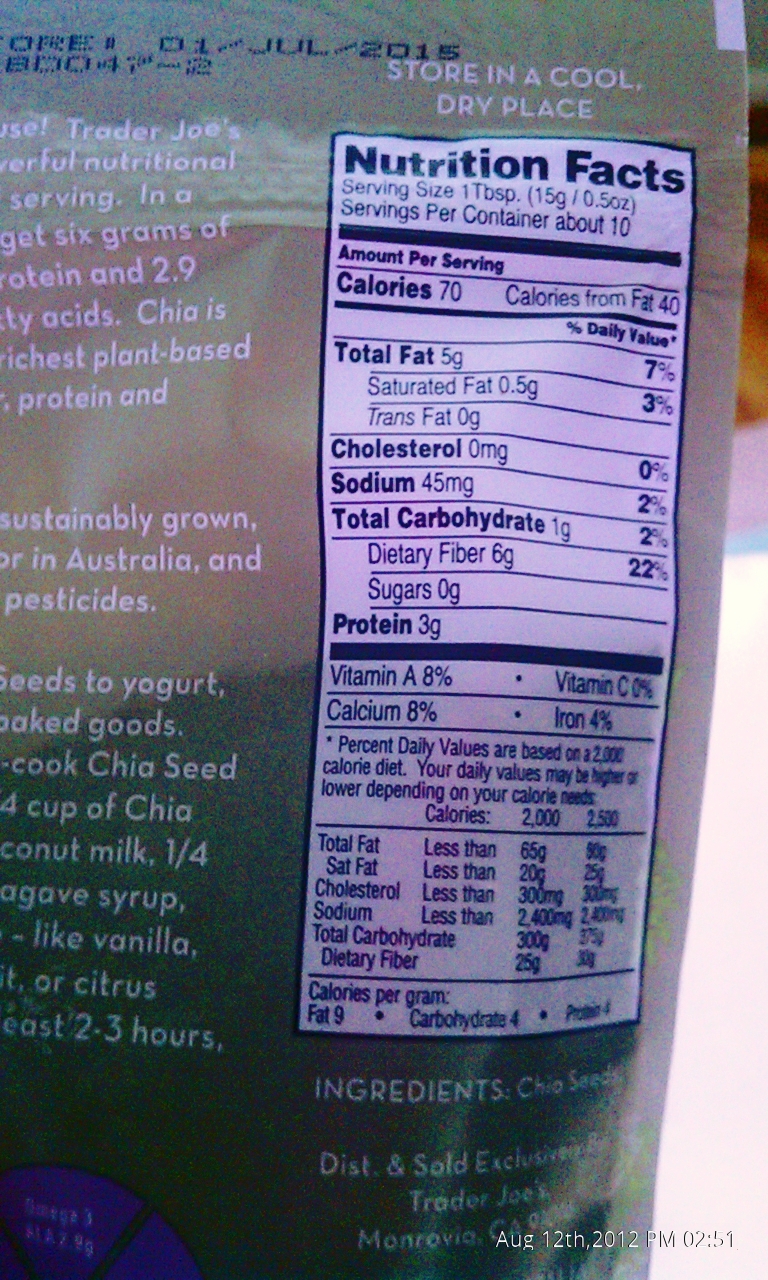The image is of the back of a Trader Joe's product package, predominantly green in color. At the top of the package, in white text, it instructs to "Store in a cool, dry place." On the top left, there is a date which appears to be the expiration date, reading "01/July/2015." 

To the right side of the package are the nutrition facts, detailing that the serving size is one tablespoon, with approximately 10 servings per container. Each serving contains 70 calories. The nutritional breakdown includes various vitamins and minerals. 

Further down, the package lists the sole ingredient as chia seeds. It also mentions that the product is distributed and sold exclusively by Trader Joe's. On the bottom left is a blue marking, while the bottom right features a watermark stating "August 12, 2012, PM 02:51." 

The background of the image includes a white platform and an indistinct brown object in the top right corner. The sides of the package contain paragraphs of text about Trader Joe's, although the full text isn't visible in the image.